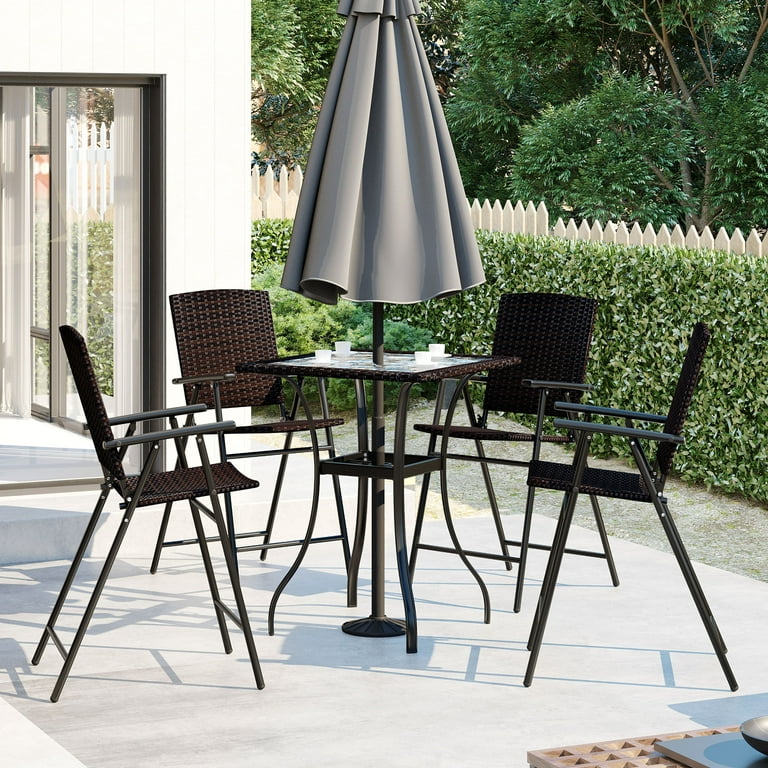The image depicts a peaceful outdoor patio area adjacent to a white-paneled house with a sliding glass door. The patio itself consists of a smooth, light-colored concrete slab. A white wooden fence with climbing vines and a row of lush bushes create a natural barrier behind the patio, with trees further in the background. The main feature of the scene is a patio furniture set, centered around a square table with a brownish, possibly glass top. An unopened gray umbrella extends from the center of the table. Surrounding the table are four high-back chairs, which resemble barstools with their tall, thin metal frames and brownish textured surfaces. The table holds four small cups. The overall atmosphere is sunny with shadows cast by the bright sunlight. An additional item, potentially a grill, is partially visible on the bottom right of the image.